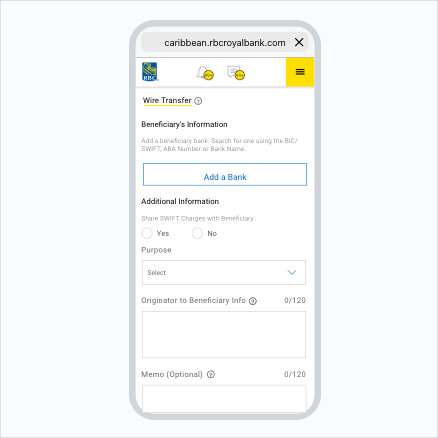This image is an illustration resembling a screenshot taken from a website, framed by the outline of a phone against a very light gray, almost off-white background. The URL displayed on the phone screen is "caribbean.rbcroyalbank.com". The screen shows the RBC (Royal Bank of Canada) website, which features a logo in the upper left corner: a blue shield with yellow accents and white text that reads "RBC".

In addition to the logo, there are several icons at the top of the page. One icon is a bell, presumably for notifications, and another is a chat bubble, likely for customer support. The content of the page appears to be a form dedicated to initiating a wire transfer. At the top, the title "Wire Transfer" is clearly visible.

The form requests several pieces of information:

- **Beneficiary's Information:** The user is prompted to search for the beneficiary's bank using a BIC, SWIFT, ABA number, or bank name. A button to add a bank is also present.

- **Additional Information:** This section includes a prompt to share SWIFT charges with the beneficiary, providing radio buttons for 'Yes' or 'No', which are currently unselected.

Other sections of the form include:
- **Purpose of the transfer**
- **Originator to Beneficiary Information**
- **Memo**

This meticulous layout indicates a comprehensive form that guides the user through the process of completing a wire transfer on the RBC Caribbean banking website.